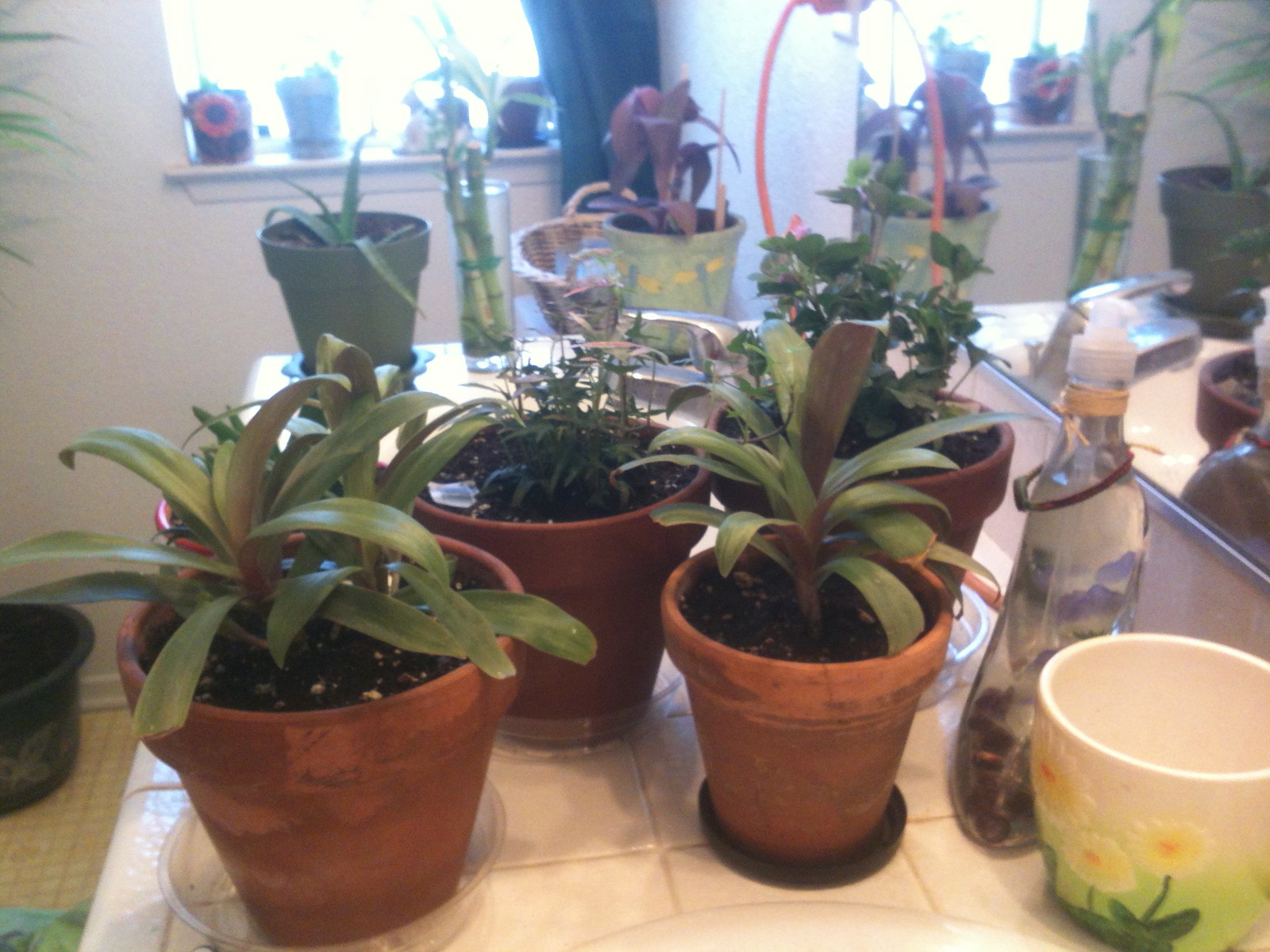The image showcases a brightly lit bathroom with a tiled counter and windowsill adorned with various plants. Most of the plants are housed in terracotta pots, with a few exceptions in green pots. In the bottom edge of the image, the rim of a sink is visible, while a cream-colored tiled counter occupies the center. A mirror is mounted on the right wall, and next to it rests a transparent soap dispenser and a decorative cup with flowers. On the left, five terracotta pots hold a variety of green plants, with some unrecognized species. Adjacent to them is a second sink, with the faucet partially visible.

Further along, a green pot holding a purplish plant is placed, and an upright clear vase with bamboo shoots is positioned in the background. Near the corner of the counter, a green pot with an aloe plant brings additional greenery. The windowsill in the background hosts more out-of-focus plants, one featuring a large orange flower. In the upper left corner, a tall plant in a base pot reaches upward. The floor is covered in small tiles, and the white walls are complemented by a blue curtain draped nearby. The photograph captures a serene and lush indoor garden space within a bright, white-tiled bathroom.